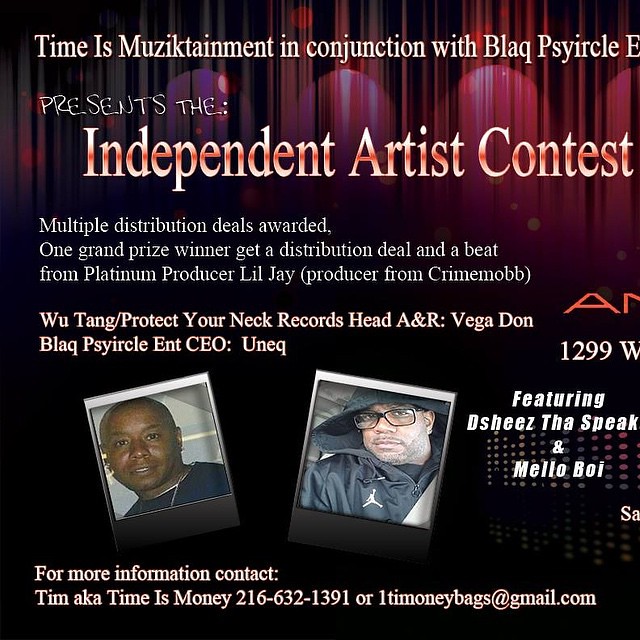This is a color advertisement with a dark black and purple background that features images of red and black stage curtains at the top. The title at the top is written in white text and says, "Time is Music Attainment in Conjunction with Blackcess." The text then gets cut off. Underneath, in bright shiny pink letters, it says, "Presents the Independent Artist Contest," followed by white text stating, "Multiple Distribution Deals Awarded." The grand prize winner will receive a distribution deal and a beat from platinum producer Lil Jay from Crime Mob. Additional information includes "Wu-Tang/Protect Your Neck Records Head A&R Vega Don" and "Black Circle ENT CEO, Unique (U-N-E-Q)." At the lower part of the image, there are photographs of two Black males, presumably the mentioned individuals, along with text featuring "D-Sheets, The Speak, and Mellow Boy." For more information, it advises to contact Tim, also known as "Time Is Money."